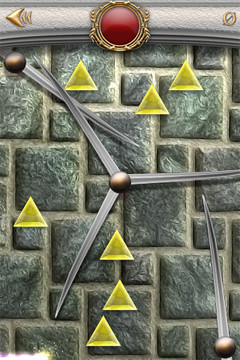The image depicts a colorful, tile-based video game interface without any visible text. The background is composed of various tiles, some are large squares while others are very small, creating a visually dynamic grid. Positioned towards the bottom of the screen, there is a mechanism designed to launch balls. This mechanism is replicated in four distinct locations: the bottom-right corner, the top-left corner, and the center. Each launching device appears to be loaded with balls ready to be propelled. Scattered strategically across the board are several yellow triangles—three at the bottom, one on the left side, and three more clustered at the top. The arrangement and design suggest a puzzle or strategy game that involves aiming and launching balls towards these triangles.